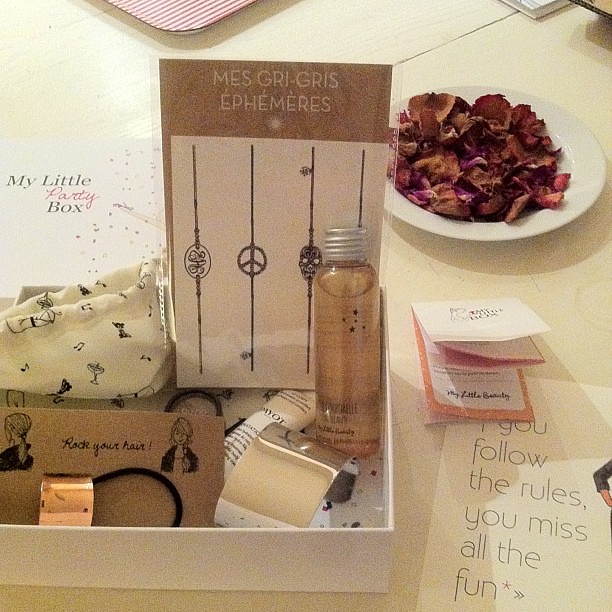The photograph showcases a well-organized dining table adorned with a variety of intriguing items. At the top right of the image, there is a dining plate garnished with a mix of dark brown, light brown, and reddish or purplish leaves, which appear to be either dried or artificial. Below this, on the bottom right, two overlapping pieces of paper can be seen; the top paper is folded into quarters with the visible flap displaying the phrase, "follow the rules, you miss all the fun," although the top word is partially cut off.

On the left side of the table, a small box labeled "My Little Party Box" is prominently displayed alongside a collection of skincare and cosmetic products. This party set includes items such as lotions, a hair twist accessory, a bracelet with a goldish reflective surface, and possibly a piece of liquid mixture in a see-through bottle with a gray cap and black star designs. Additionally, there is a white cloth goodie bag with some colorful illustrations, seemingly martinis, imprinted on it.

The table itself appears to be covered with a white tablecloth, enhancing the bright and inviting atmosphere of the scene. Some of the cosmetic items are further detailed with playful tissue paper wrapping, adding to the theme of an exciting, fun-filled surprise box experience, perfect for a little girl's party or a self-care day.